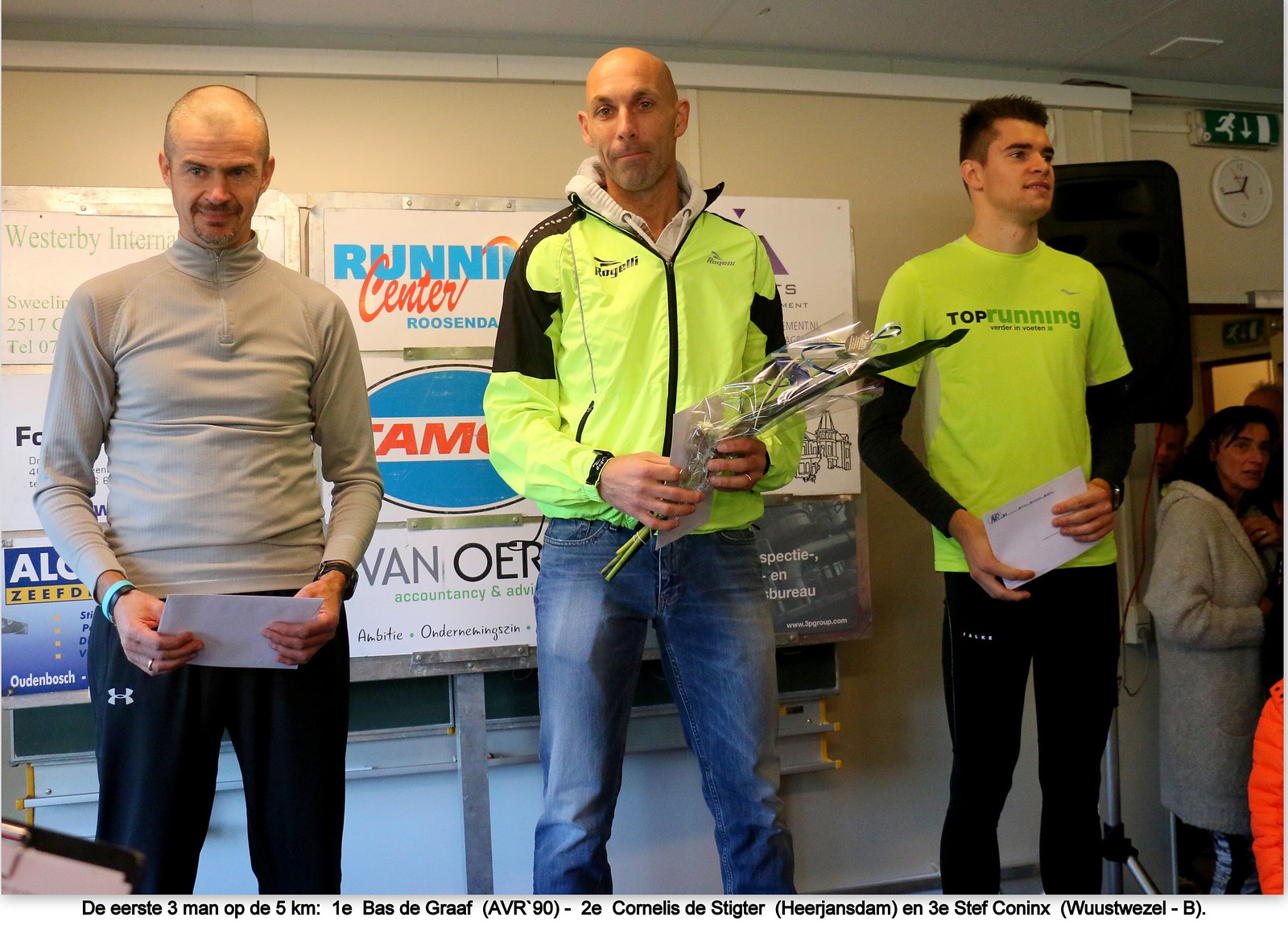In an indoor setting, likely a classroom, three men stand side-by-side before a sign adorned with various posters, the most prominent reading "Running Center Rosendale" at the top center. The man on the left, slightly balding with very short hair, dons a gray turtleneck and black Under Armour track pants, accessorized with a turquoise bracelet. The bald man in the middle sports a fluorescent yellow-green windbreaker with black accents, paired with blue jeans. He cradles a cellophane-wrapped plant or bouquet in one hand and a piece of paper in the other. The younger man on the right, with dark hair, is clad in a bright yellow shirt emblazoned with "Top Running", layered over a long-sleeve black shirt, and black running pants. All three men hold a piece of paper, indicating they might be participants or winners in a contest. Surrounding them are sponsorship logos, with a caption at the bottom of the photo that appears to be written in German.